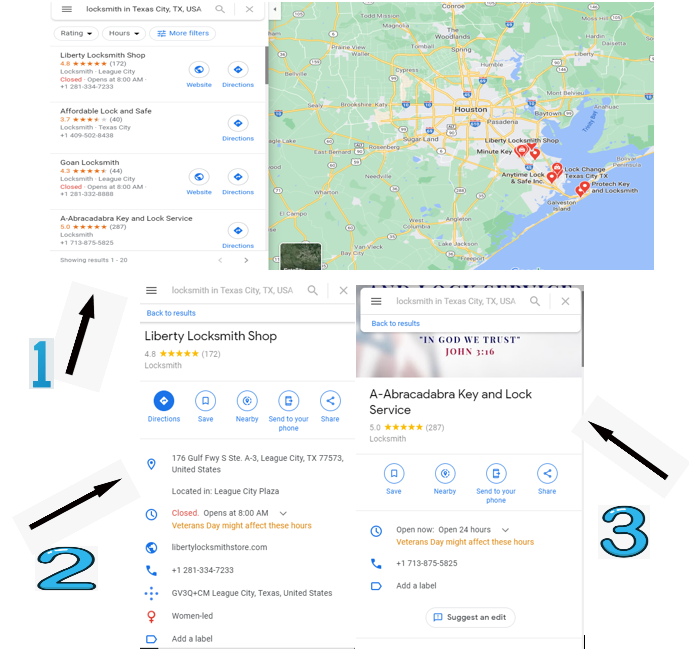The image features a collage of two Google search screenshots depicting a search for locksmiths in Texas City, Texas, using Google Maps. The first screenshot shows the search query "Locksmith in Texas City, Texas," revealing a map located slightly northeast of Houston, bordered by the Gulf of Mexico. Several locksmith businesses are marked on the map, including Liberty Locksmith Shop, Affordable Lock and Safe, Goan Locksmith, and Abracadabra Key Locksmith.

The second screenshot is a comparison between Liberty Locksmith Shop and Abracadabra Key Locksmith. Both businesses have been clicked on, displaying detailed information such as ratings and reviews. Liberty Locksmith Shop provides more detailed information about their services, but Abracadabra Key Locksmith stands out with higher overall ratings and a greater number of reviews.